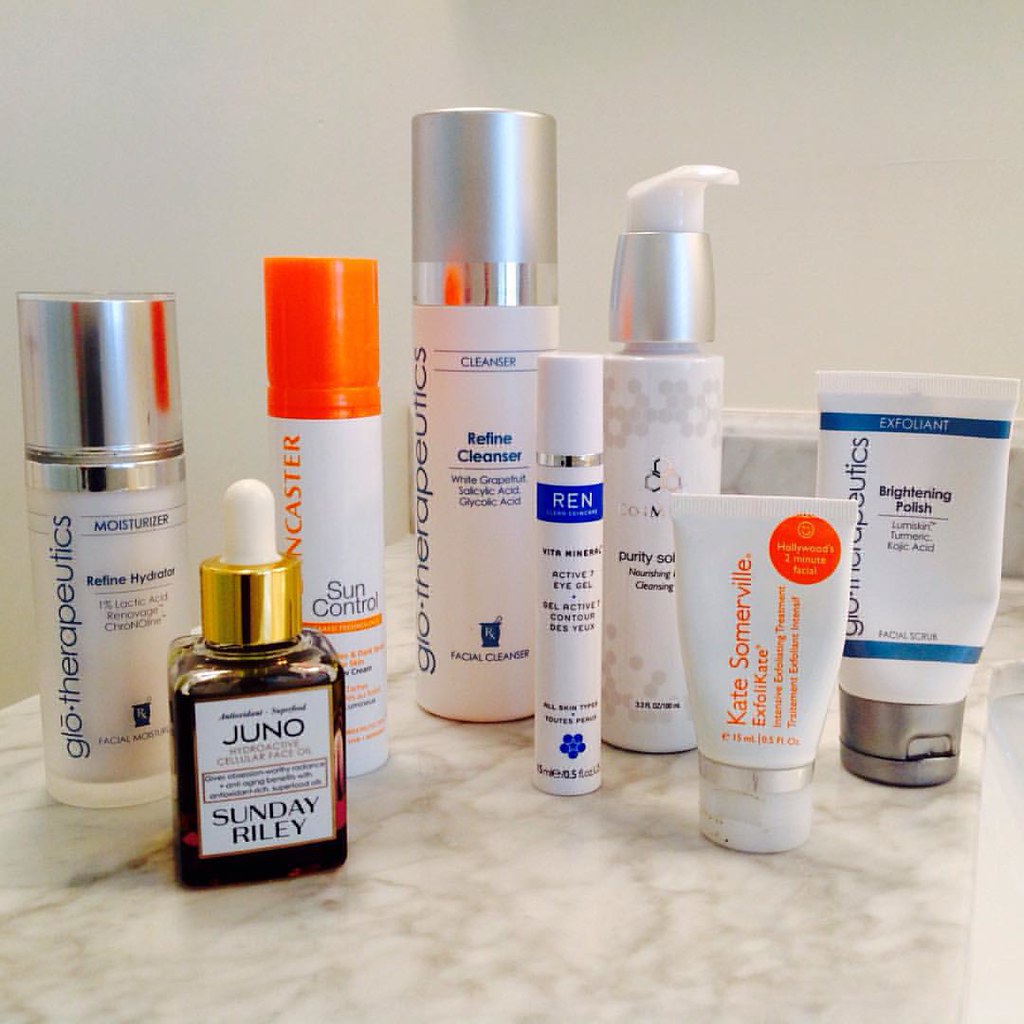In the image, we observe a relatively square area, slightly taller than it is wide by about 10%. The background features an off-white wall, occupying roughly the top half of the frame. The bottom half showcases a white marble countertop accented with light brown veining, giving it a sophisticated appearance.

On the countertop, there are eight skincare products arranged in a line from left to right. Starting from the left, the first item is a white canister with a silver top that reads "Glow Therapeutics" vertically along the side and "Moisturizer" below it. Next to it is a short, rectangular glass container with an eyedropper top featuring a gold rim, labeled "Juno Sunday Riley."

Following that, there's a tall, slender canister with an orange cap, labeled "Sun Control." The lineup continues with three more canisters and two tubes, all varied in design, suggesting a diverse range of skincare products. Each container reflects a well-organized display, indicative of a curated skincare routine.